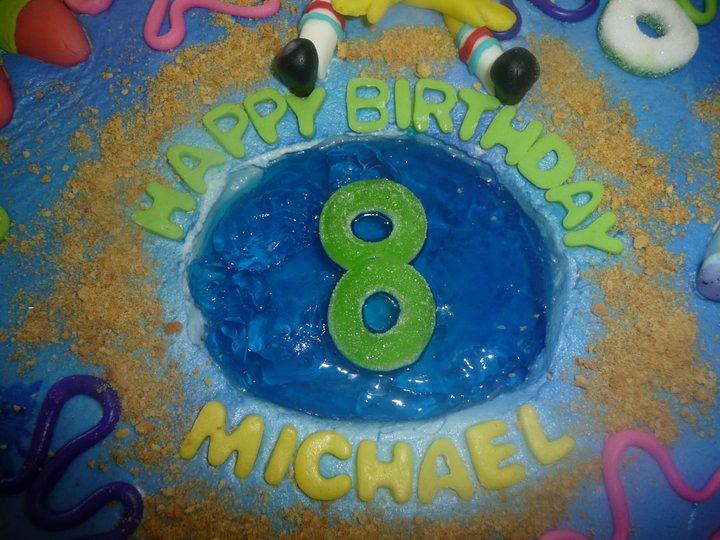This image depicts a meticulously crafted birthday cake for Michael, adorned with various confections and colorful decorations. At the center, a striking number eight, formed from two green gummy rings, rests atop a glossy blue jello-like pool. Surrounding this focal point, light blue icing spreads across the cake, accentuated by scattered brown sugar or graham cracker crumbs.

The celebratory message, "Happy Birthday" in green gummy letters, arches gracefully across the upper section, while "Michael" is prominently displayed below in bright yellow. The edges of the cake feature intricate details, including purple and pink squiggly lines of writing icing in the bottom left and right corners, respectively, and similarly colored detailing along the top.

To complete the scene, the top decoration includes characters resembling Patrick and SpongeBob from the beloved cartoon show, with their legs and feet crafted from icing. Patrick's signature pink squiggly legs and SpongeBob's distinctive black shoes, white socks, and striped accents are positioned around the cake, adding a whimsical touch to this celebratory centerpiece. The top right corner intriguingly displays an upside-down white donut or apple ring, enriching the cake's textural variety.